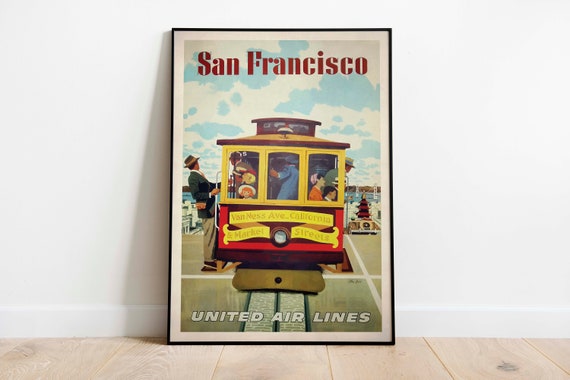The scene depicts a bright, minimalist room featuring a light tan, wide-planked wooden floor, and a stark white wall with white trim. Leaning against the wall is a rectangular poster in a black frame, prominent in the middle of the image. The poster casts a slight shadow to the left side. At the top of the poster, the red text reads "San Francisco," set against a blue sky with white clouds. Below, a red and yellow cable car labeled "Van Ness Avenue, California, Market Streets" occupies the center. The cable car is bustling with various individuals, including a man in a brown hat, brown pants, and a blazer hanging off its side. An Asian woman is visible on the right side of the trolley. The bottom of the poster features bold white text that says "United Airlines."